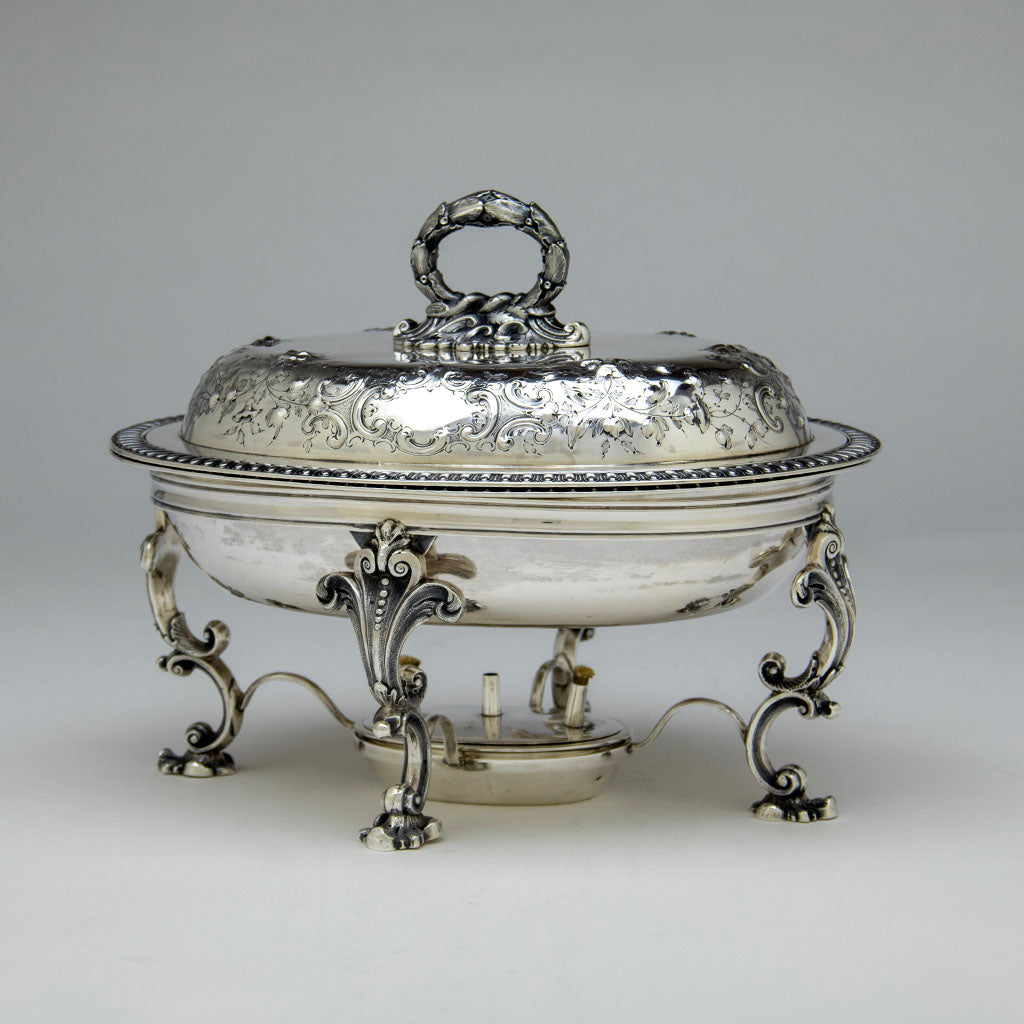The image showcases a close-up of an antique Rococo-style silver chafing dish, resting on a whitish-gray background that darkens towards the top. The oval, bowl-shaped platter features four ornate, tiny legs, each intricately crafted. The dish includes a bottom section designed to hold a heat source, ensuring the food inside stays warm. The rim is adorned with detailed dental engravings, enhancing its elegant appearance. The silver cover of the dish boasts elaborate floral and ornate Rococo engravings, crowned with a decorative handle shaped like an organic figure, adding to the overall ornate craftsmanship of the piece.